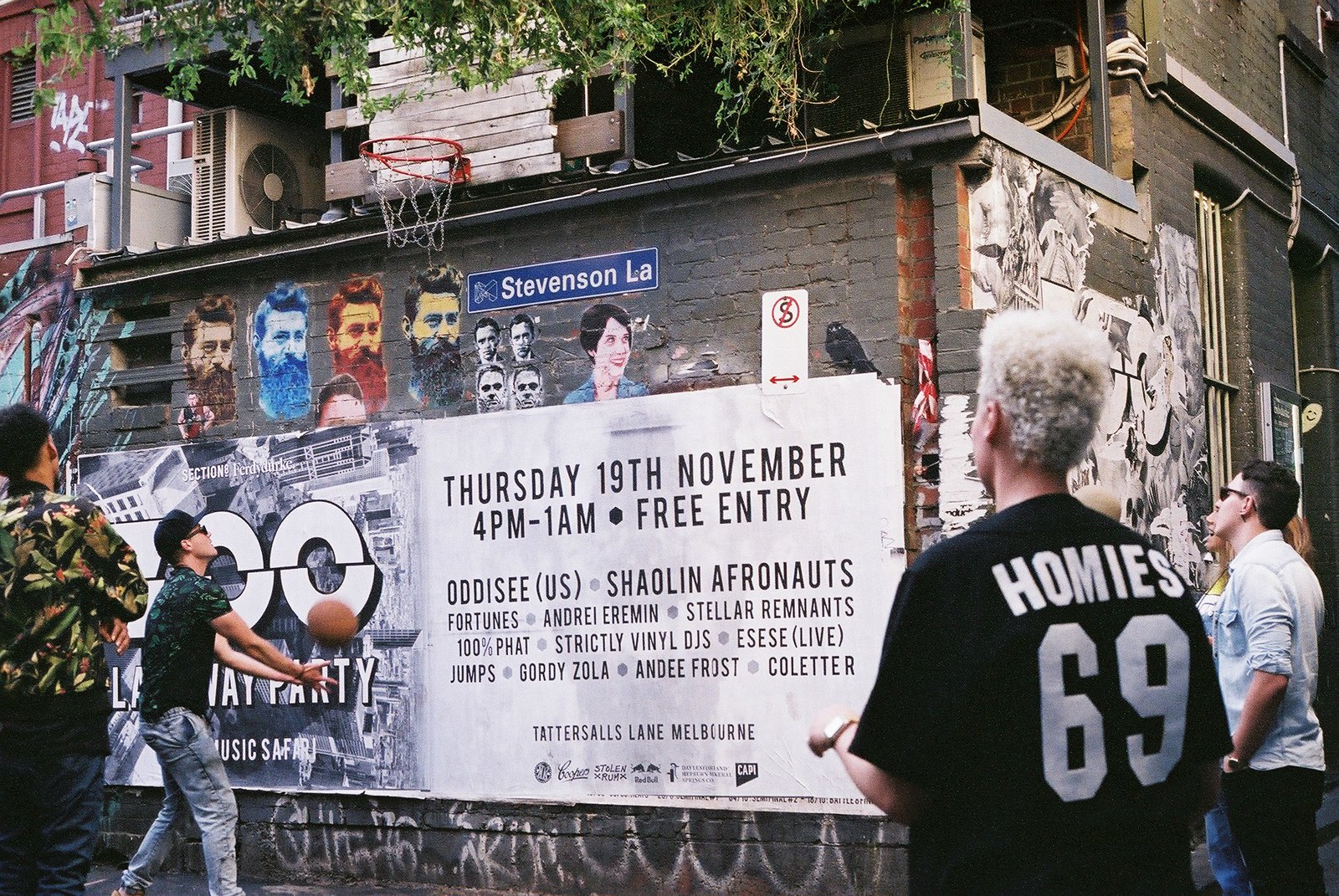In this detailed outdoor scene, an image captures a casual basketball game set in front of a large, gray-wall brick building adorned with various posters and graffiti art. Prominently displayed is a red basketball hoop mounted against the wall. Surrounding the scene are four men engaged in the moment. The man closest to the hoop is mid-action, shooting the basketball with both hands. He is wearing a black button-up short-sleeved shirt, jeans, and a backward black baseball cap. To the right, an older white man with white hair, dressed in a black t-shirt emblazoned with "Homies 69" on the back, observes the game intently. Another observer, positioned further back, sports a short-sleeved white button-up shirt and sunglasses. On the left side of the frame, partially cut off, stands a fourth man wearing a floral-patterned shirt and black pants, with his arms folded across his chest. The building's wall features a colorful variety of graffiti, showcasing images of a bearded man in different hues such as orange, blue, brown, and a tan-black-and-white mix. There's also a painting of a woman and smaller forehead portraits. A centrally placed sign on the wall announces an event: "Thursday, 19th November, 4 pm to 1 am, free entry" along with the names of multiple artists and DJs spanning across genres, suggesting a vibrant urban setting in Melbourne's Tattersales Lane. The ground is an asphalt surface, typical of city play areas, and the atmosphere is lively yet casual, with elements of urban art contributing to the dynamic backdrop.